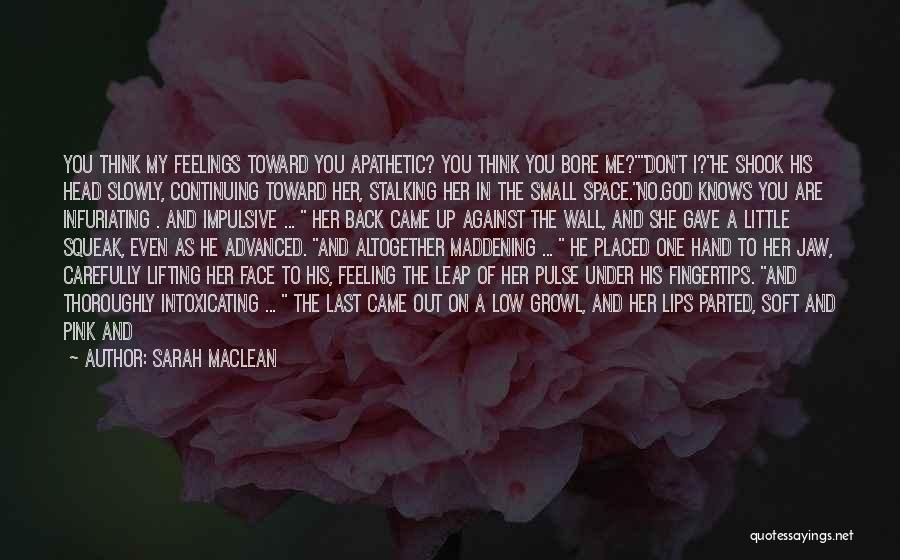The image features a large, muted pink background with green edges, accented by a subtle design of faded flower petals. At its center, in bold white or yellow capitalized font, is a striking quote that reads: "You think my feelings towards you apathetic? You think you bore me, don't I? He shook his head slowly, continuing toward her, stalking her in the small space. No, God knows you're infuriating and impulsive. Her back came up against the wall and she gave a little squeak even as he advanced. And altogether maddening, he placed one hand to her jaw, carefully lifting her face to his, feeling the leap of her pulse under his fingertips and thoroughly intoxicating. The last came out on a low growl and her lips parted, soft and pink..." The quote is credited to author Sarah McLean, with "Quotesayings.net" marked in small font at the bottom right corner. The composition emphasizes the intensity and emotional depth of the words, designed to be impactful and shareable on social media platforms.